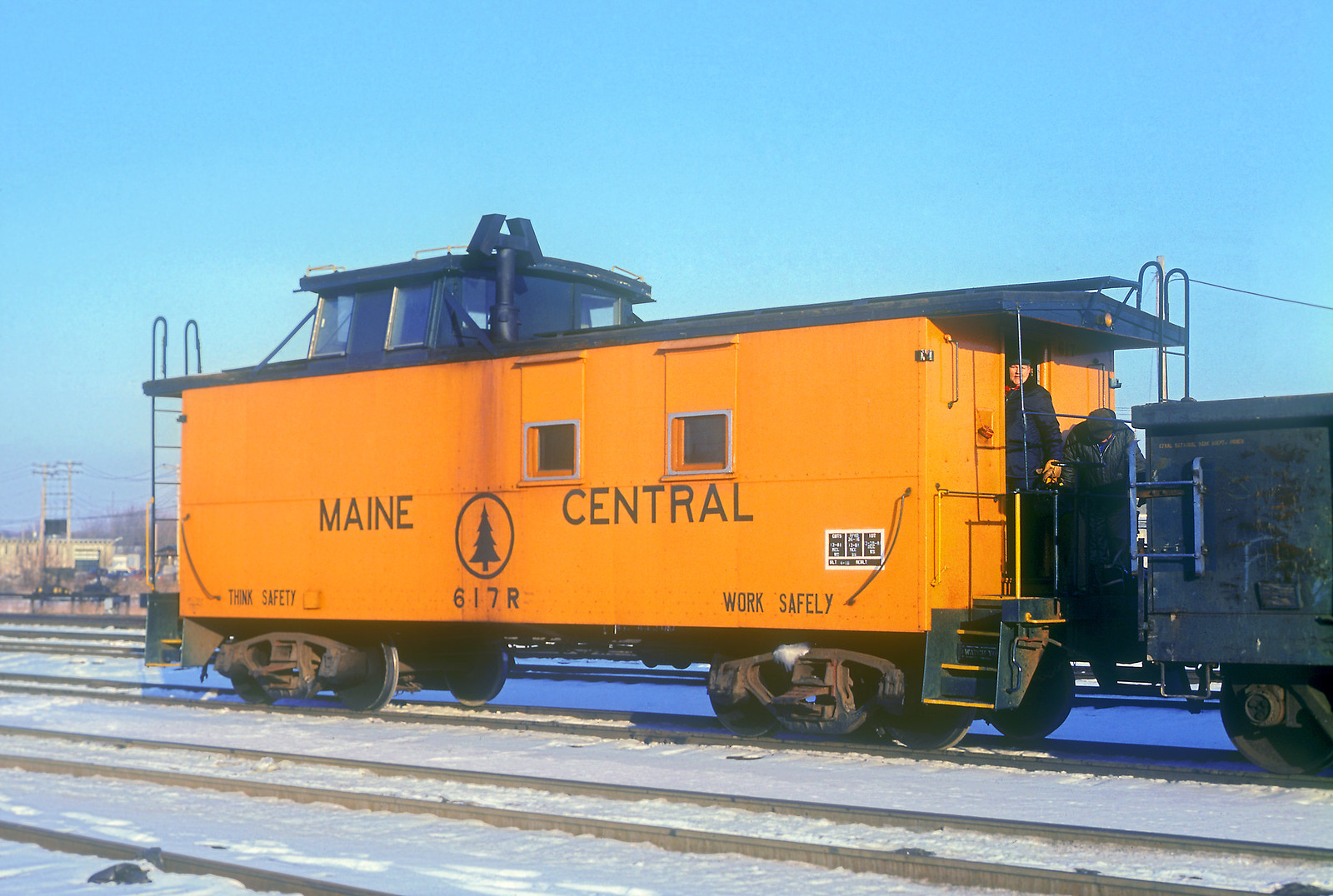This is an image capturing a winter scene of a train car on snowy tracks under a clear blue sky. The train car is a deep school bus yellow with black trim, black wheels, and is connected to another black train car in front of it. This rail car, serving as the engine, is marked with "Maine Central" in bold letters, along with the safety motto "Work Safely, Think Safety" and the number "617R." A circle icon housing a pine tree is also displayed on its side. Additionally, there's a prominent elevated cockpit with windows on top of the car, reminiscent of a lookout.

Two older white men, dressed warmly in dark blue or black coats, gloves, and hats, are visible. One man looks down while the other gazes directly at the camera. These men are likely the train's operators. In the background, power lines, a few trees, and some buildings are visible, emphasizing the frigid, open landscape. The overall scene exudes a sense of quiet but purposeful industry amid the cold winter day.